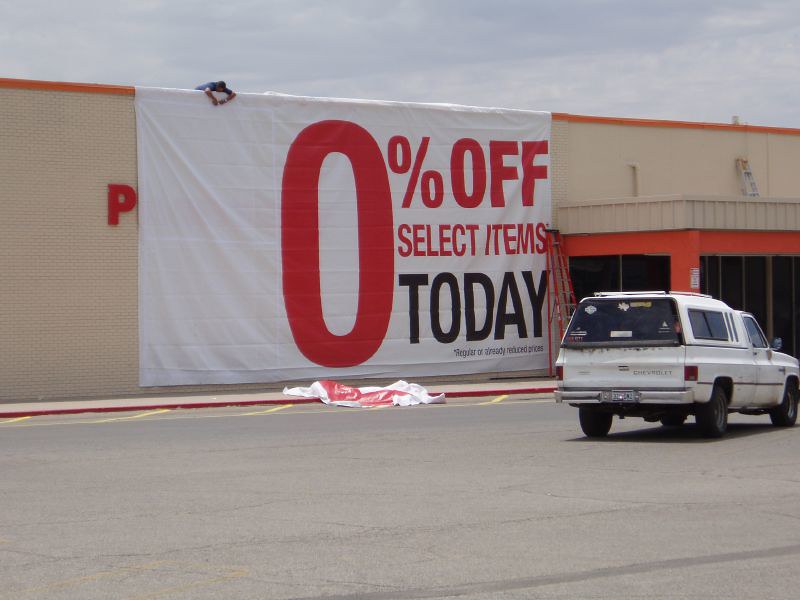The image showcases a bustling loading zone clearly marked by white lines on a large gray asphalt floor. Dominating the right side is a white truck that resembles a hearse, sporting a large truck bed and adorned with numerous stickers on its rear window. The truck prominently displays the Chevrolet brand name and has a visible license plate. To the far right, shadows cast a darker hue. On the left, a sturdy wall made of white bricks stretches upwards, adorned with red lettering.

Atop this wall, a person leans over a fabric banner that drapes down, displaying bold red text reading "0% off select items today," with some finer print also present. The sky overhead is filled with gray clouds, adding a somber tone to the scene. Adjacent to the banner is a structure comprised of white or off-white elements contrasted by red components, possibly indicating an entryway. A striking red ladder is propped up against the wall, extending towards the fabric banner. Finally, the sidewalk in the foreground boasts a distinguished red curb, adding a splash of color to the monochromatic setting.